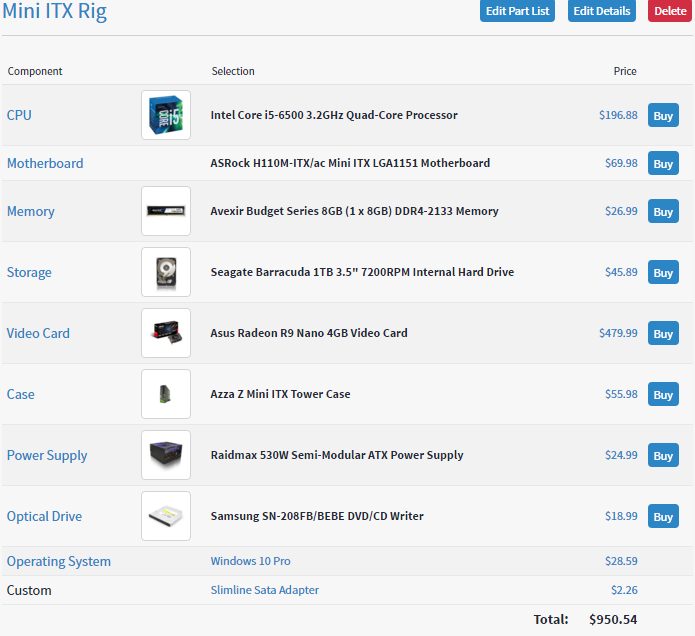Screenshot of an ITX rig build with detailed component list and pricing. The image displays various options such as "Edit Part List," "Edit Details," and "Delete," along with sections for component selection and prices. The highlighted components include:

- **CPU**: Intel Core i5-6500, 3.2GHz Quad-Core Processor priced at $196.68. The CPU selection is marked in blue.
- **Motherboard**: ASRock H110M-ITX/AC Mini ITX LGA1151 priced at $69.98.
- **Memory**: Avexir Budget Series 8GB (1x8GB) DDR4-2133 priced at $26.99.

The screenshot showcases the structured layout for building an ITX rig with specific components and associated costs.